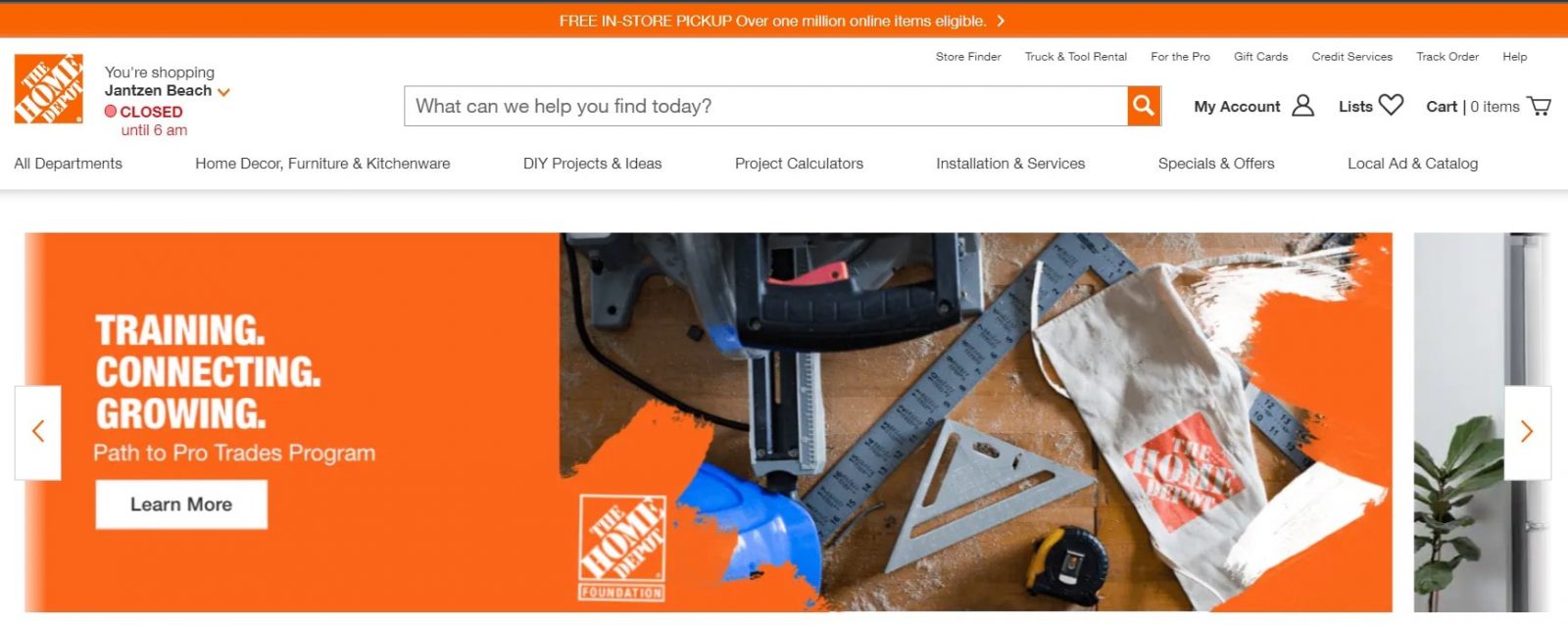The image is a screenshot of a website, specifically from The Home Depot. At the very top, a prominent bright orange banner stretches across the width of the page, featuring centered white text that reads, "Free In-Store Pickup Over 1 Million Online Items Eligible," with an arrow pointing to the right, indicating further information or a link.

Below the banner, the background transitions to white. In the upper left corner, there is an orange square with "The Home Depot" written in white text inside it. Just outside of this square, the text reads, "You're shopping Janssen Beach," accompanied by a downward arrow, followed by red text stating, "Closed until 6 a.m."

Centered on the white background is a bold prompt: "What can we help you find today?" directly above a search bar. To the right, the interface displays "My Account" and a list indicating "0 items" in the cart, depicted by a shopping cart icon.

The navigation menu allows users to browse various categories, including "All Departments," "Home Decor," "Furniture & Kitchenware," "DIY Projects & Ideas," "Project Calculators," "Installation & Services," "Specials & Offers," and "Local Ad & Catalog."

Further down, the page transitions to a section with a background that has an orange accent on the left side. This section is dedicated to the "Path to Pro Trades Program," with a heading that reads "Training. Connecting. Growing." Beneath this, it says "Learn More." Various graphics enhance this section, displaying tools such as hard hats, measuring tapes, and an apron, signifying the trades and hands-on projects promoted by the program.